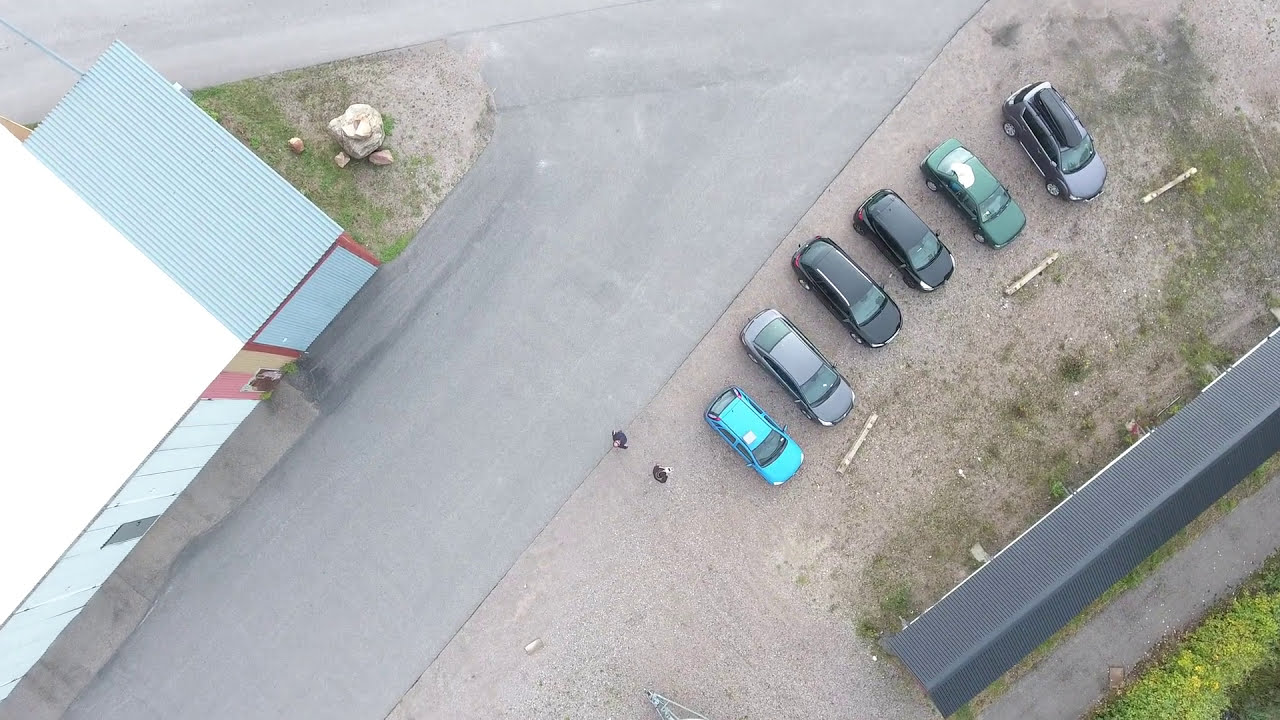This is an aerial daytime photograph showcasing a diagonal stretch of a grey road devoid of vehicles in the center, with diverse elements on either side. To the right of the road, there is a light brown ground area hosting a total of six parked vehicles, variously colored in hues like dark green, black, and one with a turquoise hood and top. Near these cars, two individuals can be seen standing. On the upper right, one of the cars has a carrying container, possibly for skis. The ground here is a mix of gravel and paved sections. On the left side of the road, there's a large, almost cuboidal building characterized by a white and blue roof made of light bluish turquoise metal. Adjacent to this building, there is a grassy area with a large rock. The overall setting captures a real view of a roadside area within a horizontal rectangular frame.